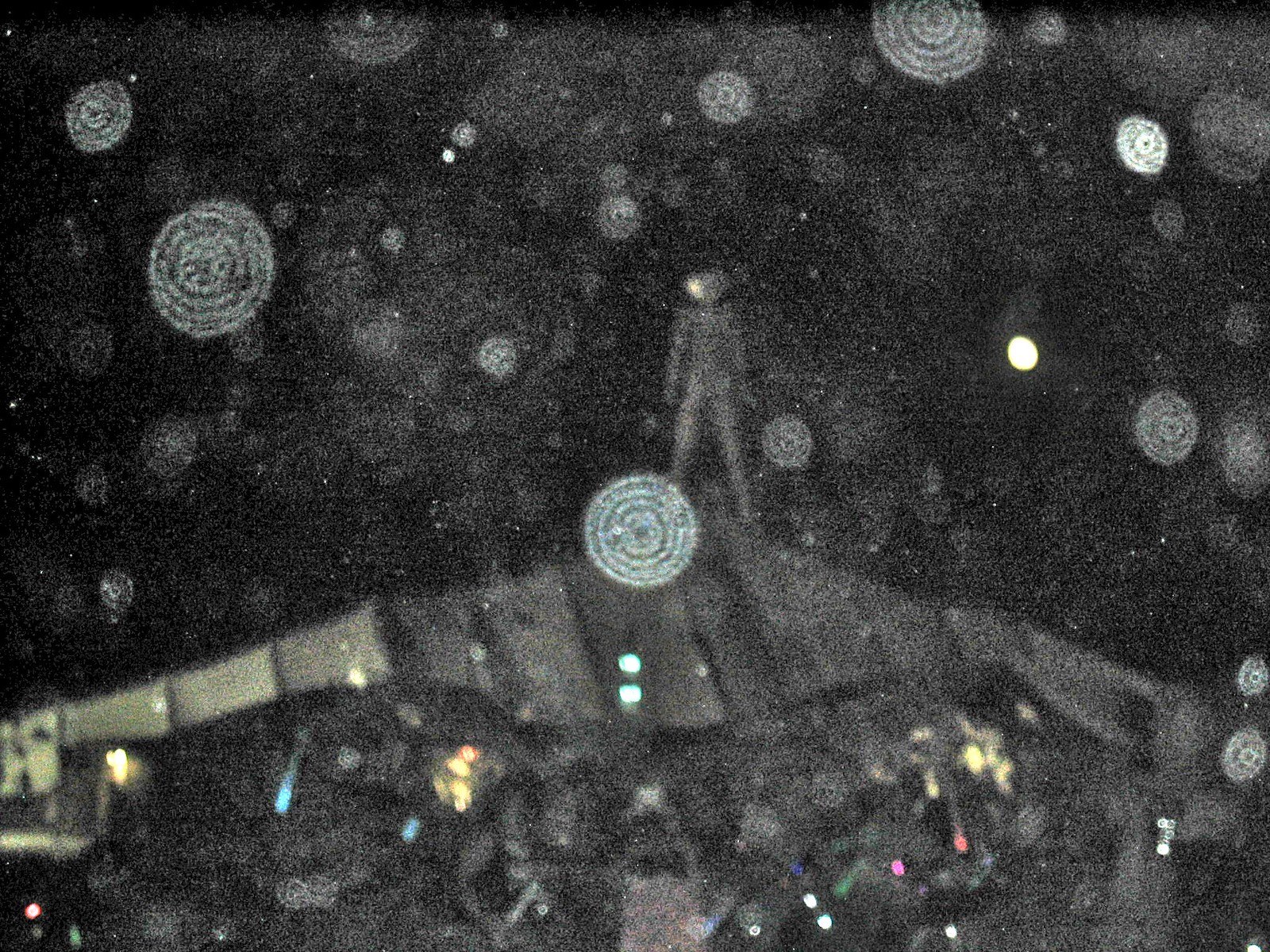In this image, a dark and enigmatic scene unfolds, seemingly designed by AI or created through computational artistry. Dominating the composition is a humanoid figure with a human-sized frame, standing on a metallic hilltop. The figure's head is visible, but its face is obscured, adding to the mysterious atmosphere. Large, translucent rocks with diamond-like qualities are scattered in the foreground, showcasing subtle color refractions that glimmer and shift as if catching faint light. The entire scene is punctuated by numerous light splotches, which contribute to the surreal and otherworldly ambiance of the artwork.